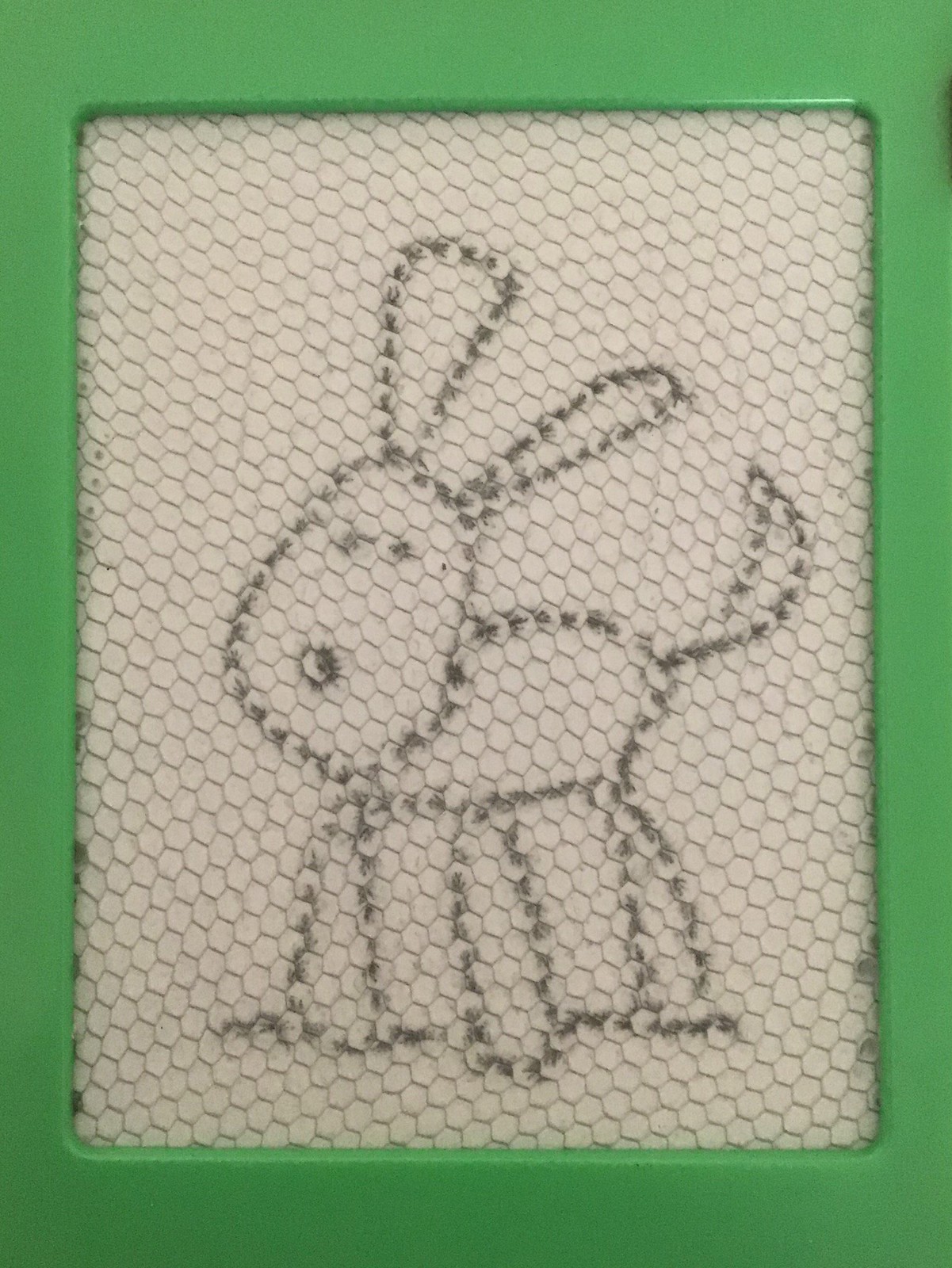The image depicts a playful stick figure dog sketched on a classic magnetic drawing board with an attached stylus. The dog features tall, floppy ears and a small black nose that adds a touch of character to its simplistic design. Its tail appears to be wagging, suggesting a sense of motion and excitement. The dog's legs are rendered as stick figures, which contrasts with the more detailed depiction of its ears and tail. Besides the green border framing the magnetic drawing board, the entire illustration is presented in black and white, emphasizing the minimalistic yet charming nature of the artwork.